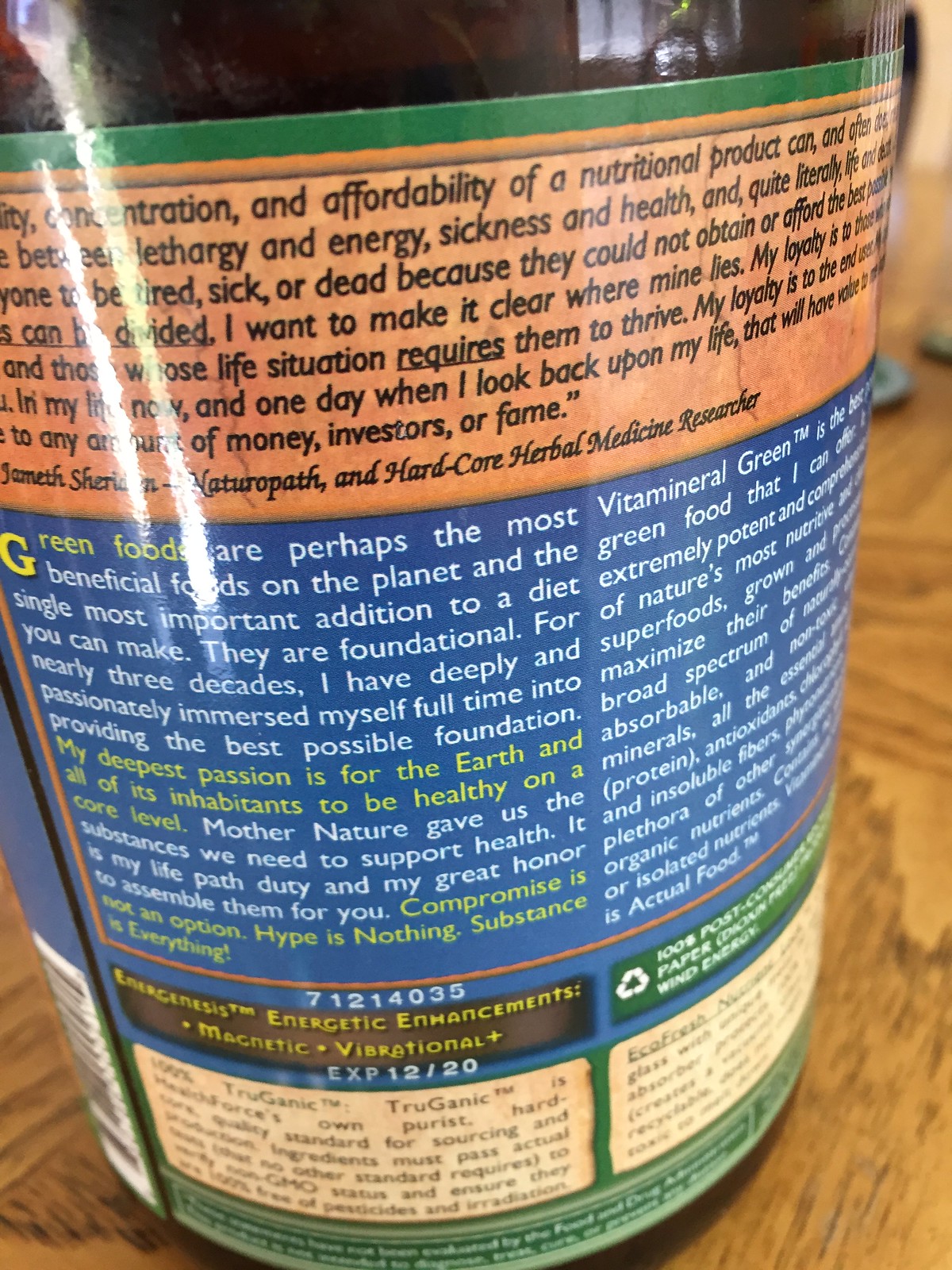This close-up photo displays the side of a label on a cylindrical brown bottle, likely made of glass or plastic, sitting on a wooden table. The label is from the brand Truganic™, and it's packed with detailed information arranged in three main sections. The top section features an orange background with black text, which includes a quote attributed to Janeth Sheridan, a naturopath and hardcore herbal medicine researcher. This section is partially cut off in the photo.

The central section has an eye-catching blue background filled with white text. Here, a statement emphasizes the unparalleled benefits and foundational importance of green foods, asserting they are the most crucial addition one can make to their diet. Despite the extensive content, the legible parts include the passionate dedication of the author, who has spent nearly three decades immersed in providing top-quality products. Yellow text interspersed within the white adds emphasis to certain key points, including a dedication to health and a declaration that compromise is not an option while hype is worthless; substance is everything.

Adjacent to this blue section, curving around the bottle, is an additional paragraph of white text, further elaborating on the product's virtues. The bottom section of the label features an off-white or parchment-like background with black text, though this part is somewhat blurry and tough to decipher. Several other elements, like green and brown-colored individual boxes, a brown box with yellow text reading "Energenesis" and "Magnetic Vibrational Enhancements," and a white barcode, contribute to the label's vibrant and information-rich design.